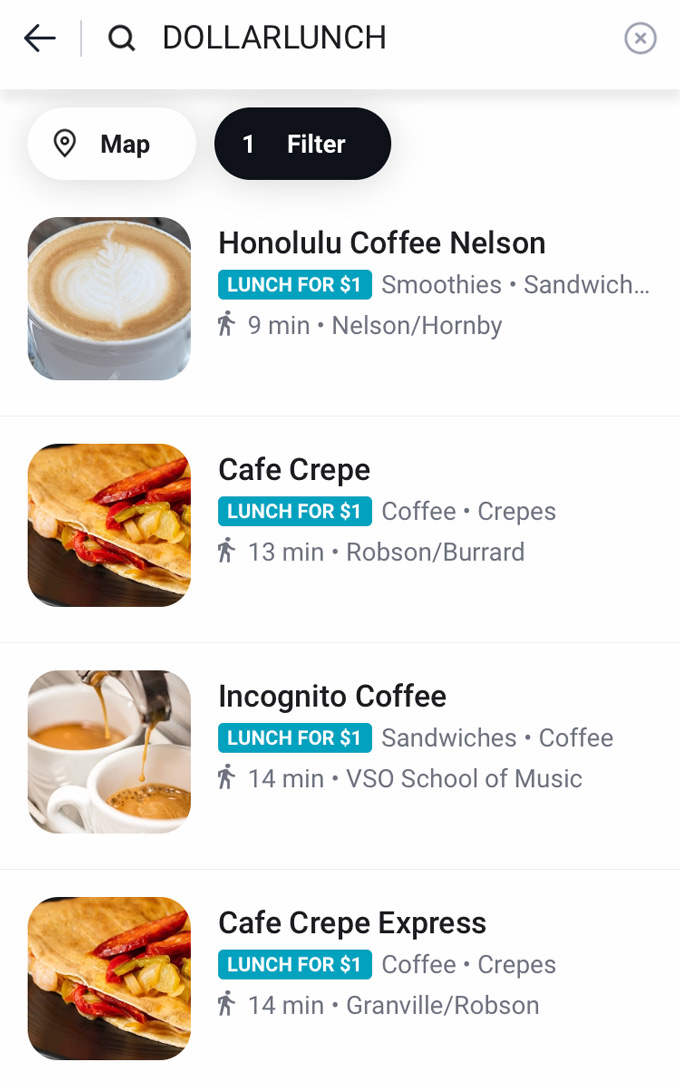Screenshot of a food delivery app interface highlighting a "Dollar Lunch" search result. At the top, the header displays "Dollar Lunch" alongside a search bar, with a back arrow on the left and an 'X' to close on the right. Below the header, there are interactive buttons including a white button labeled "Map" with a pin drop icon to the left, and a "Filter (1)" button in black indicating an active filter.

The main section lists various businesses each tagged with a "Lunch for a Dollar" banner in blue. For instance, the first entry is "Honolulu Coffee Nelson," showcasing their offerings listed in gray text to the right of the blue banner. The specifics include "Smoothies" and "Sandwiches." Additionally, at the bottom of this entry, there is an icon of a walking person beside "9 minutes," indicating the walking distance, followed by the tag "Nelson Hornby" for the area.